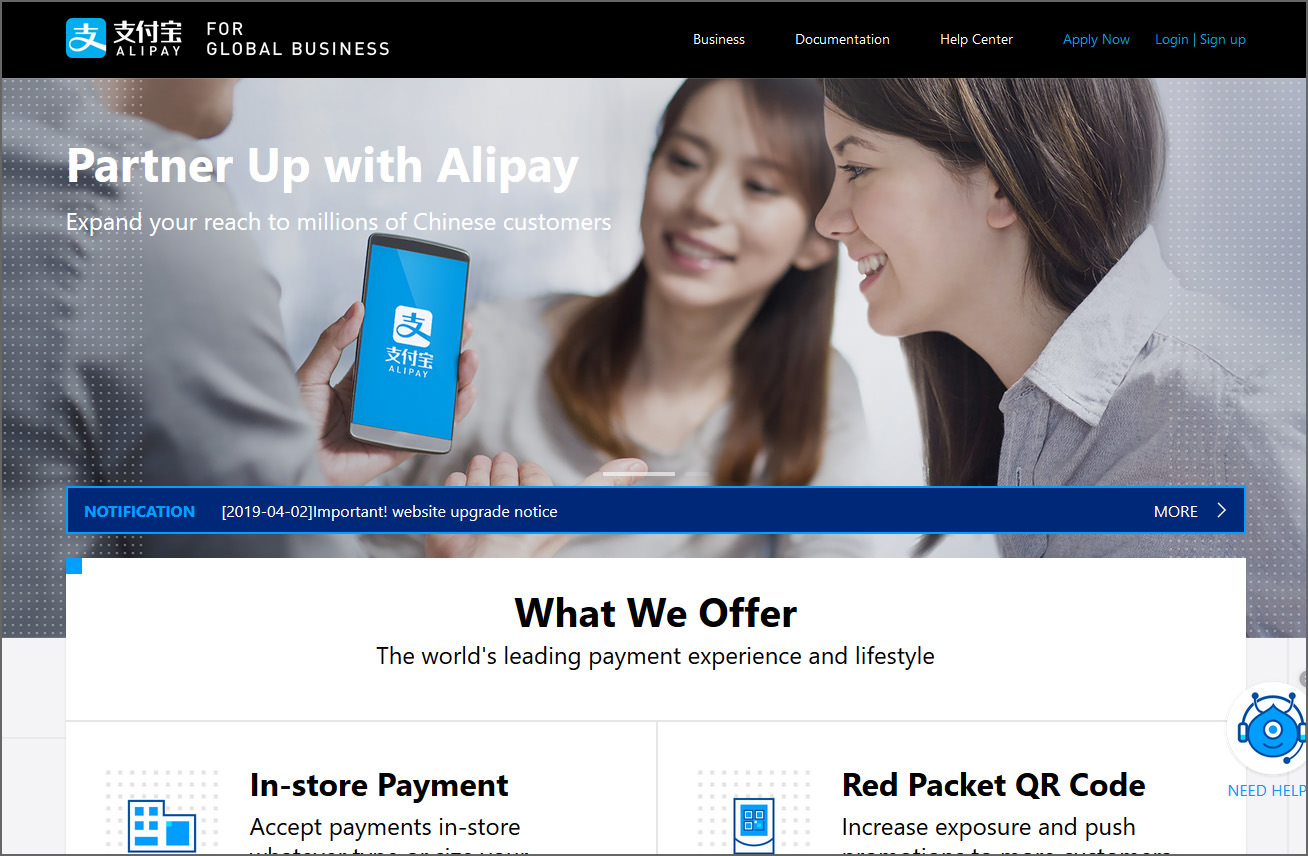Screenshot Description: Alipay Advertisement

This screenshot showcases an advertisement for Alipay, primarily targeted at global businesses. The interface features a header with multiple navigation options, including "Business," "Documentation," "Help Center," "Apply Now," and "Login/Sign Up." Adjacent to the phrase "for global business," there is Chinese text.

Below the header, the advertisement displays an image of a man holding up a cell phone, which captures the attention of two women. All three individuals are dressed in white and have brown hair. The scene suggests a moment of shared interest or a demonstration of the Alipay app.

Underneath this image is a notification banner dated April 2, 2019, reading "Important website upgrade notice," with an arrow indicating more information is available.

Further down the page, a section titled "What We Offer" describes Alipay as providing "the world's leading payment experience and lifestyle." This section introduces two key services: "In-Store Payment," which encourages merchants to accept payments in-store, and "Red Packet QR Code," promoting its utility to increase exposure and push notifications.

At the bottom right-hand corner of the screenshot, there is a button featuring an icon of a bug with headphones, labeled "Need Help," likely a portal to customer support services.